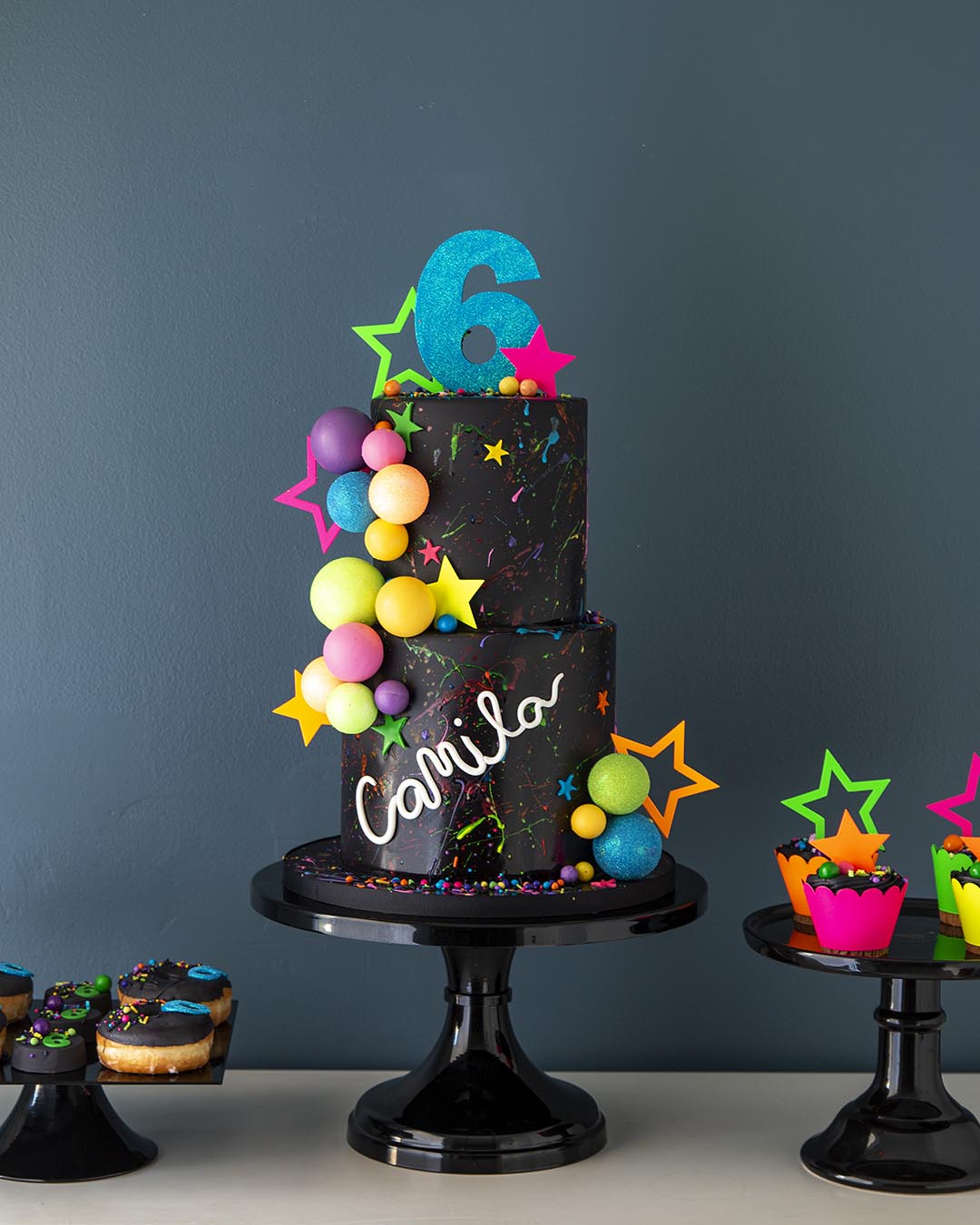This photograph captures a vibrant and meticulously arranged birthday celebration display for a girl named Camilla on her sixth birthday. It features three platform cake stands aligned horizontally on a cream-colored table. The first stand, small and squat with a flat square surface, supports a tempting assortment of chocolate-frosted doughnuts adorned with colorful icing. Centrally positioned is the largest black cake display stand, featuring an impressive two-tiered black cake. The bottom tier is a tall, cylindrical base about six to seven inches high, topped by a smaller cylinder of about four to five inches. A prominent blue number six decorates the cake's peak. The cake itself is festooned with an array of neon-colored balls and stars in shades of green, orange, yellow, purple, and pink, creating a striking contrast against the black frosting. Diagonally written in white cursive icing on the cake is Camilla's name, C-A-M-I-L-A, adding a personalized touch. The right-most stand, medium in size, displays an array of multicolored cupcakes that echo the neon theme. This elaborate and visually striking setup vividly highlights the joyous occasion of Camilla's sixth birthday.